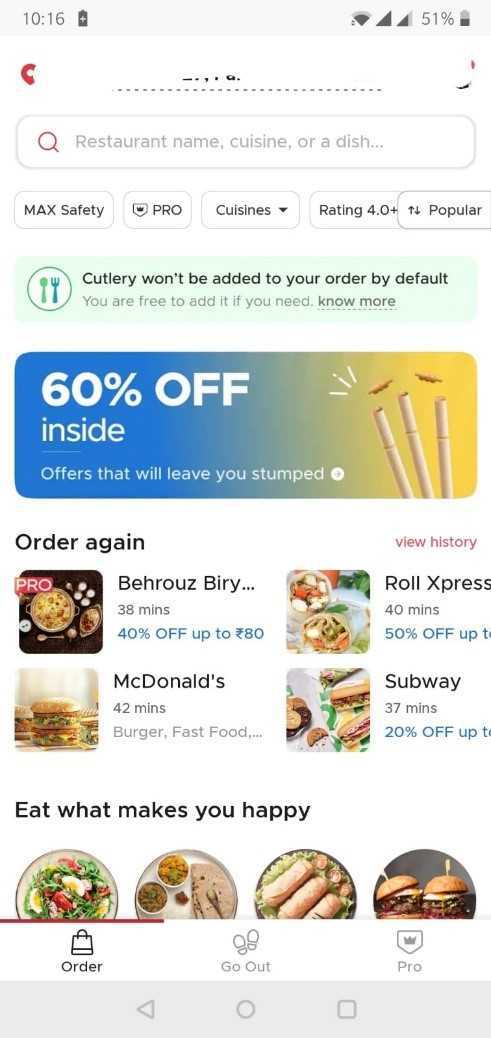The image is a screenshot of the DoorDash app interface. At the very top, the recognizable DoorDash logo is prominently displayed. Below the logo is a search bar where users can input restaurant names, specific cuisines, or dishes they wish to find. Directly beneath the search bar, there are several clickable suggestions for quick searches including options like "Mac Safety," "Something Pro," "Cuisine," "Rating 4 or Higher," and "Popular."

Further down, a notification informs users that cutlery will not be added to their order by default, although they have the option to add it if needed. A clickable note labeled "No More" likely offers additional information on this policy.

The next section highlights a promotional deal titled "60% Off Inside," which is accompanied by an image that seems to depict bamboo, though the exact nature of the image is unclear. 

Following the promotional section is an "Order Again" feature, which lists restaurants the user has previously ordered from. Next to each restaurant, current offers are displayed: Behrouz Biryani offers 40% off on orders over $80, Roll Express provides 50% off, and Subway has a 20% discount available.

At the bottom of the page, there's a motivational message: "Eat What Makes You Happy," accompanied by additional suggestions for the user to explore.